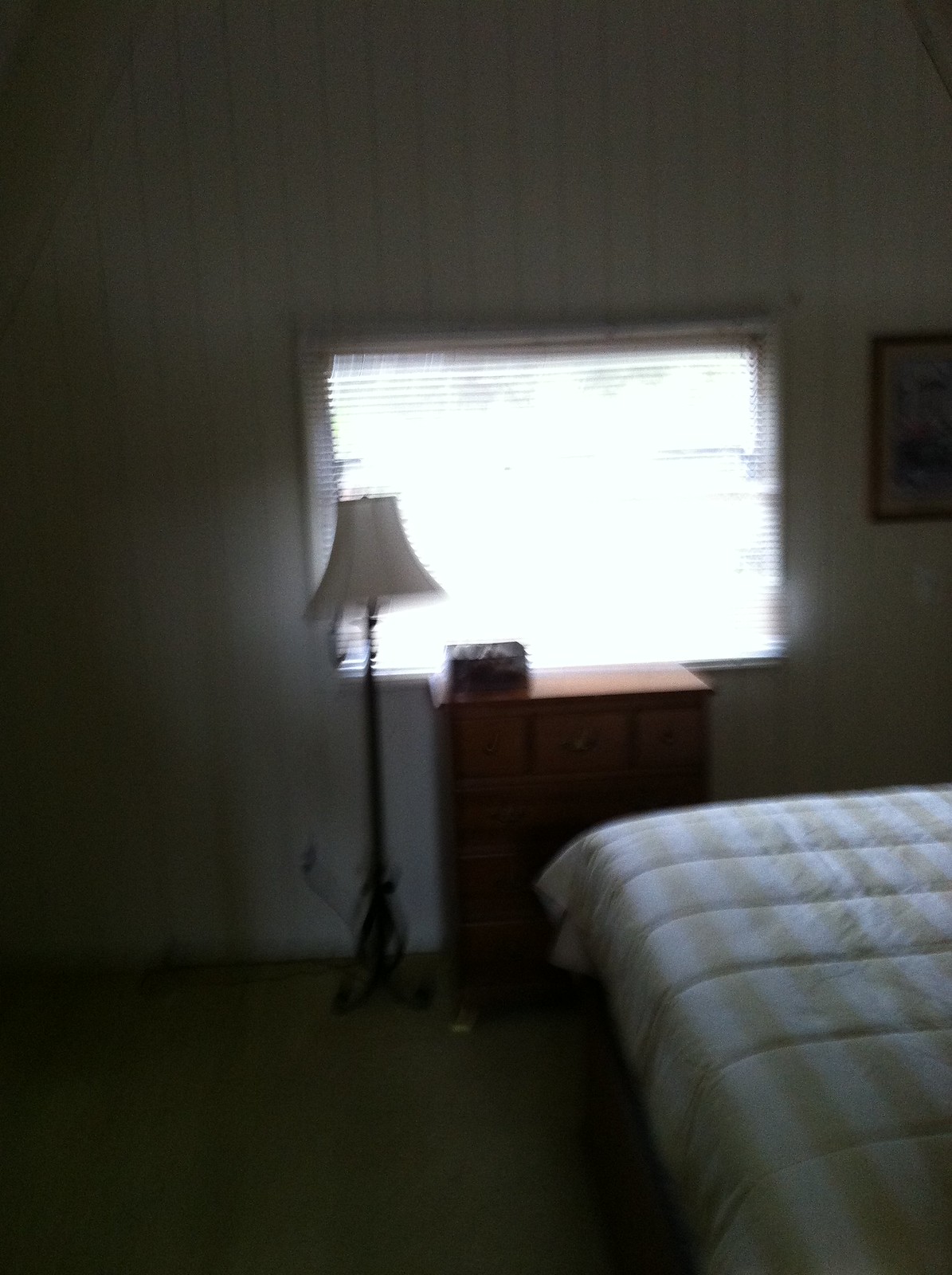The image depicts the interior of a bedroom with a somewhat blurry quality. The flooring appears to be made of a cheap material, possibly gray concrete. The wall behind the main features of the room is white and consists of long, parallel wooden strips, painted white. A window with blinds dominates the wall, allowing an abundance of natural light to flood the otherwise dark room, creating a stark, glowing rectangle effect.

In front of the window, a lamp with a curled base and a white lampshade stands on the floor. Nearby, there's a wooden dresser with an unspecified box resting on top of it. On the right-hand side of the image, part of a painting with a brown wooden frame is visible. In the bottom right quadrant, a bed is seen with a white bedspread adorned with pale yellow stripes.